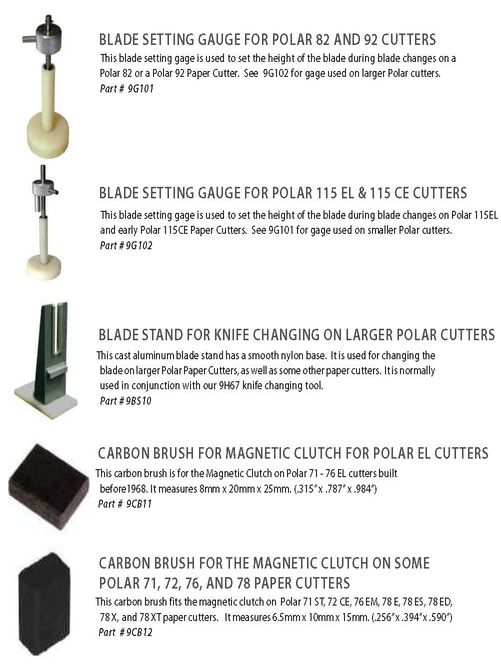The image is a detailed infographic resembling a parts catalog for components used in paper cutting machines. It is set on a white background with black text and contains five product images, each associated with a description and part number. The products include a blade setting gauge for Polar 82 and 92 cutters, another gauge for Polar 115 EL and CE cutters, a blade stand for safe knife changing on larger cutters, and two carbon brushes, one for a magnetic clutch in Polar EL cutters and the other for various Polar paper cutters. Each item is depicted in various colors with the image on the left and a concise description on the right, specifying the part's appearance, dimensions, and usage details. The blade stand is described as having a base with a slotted gray shape to assist in blade changes, while the carbon brushes are dark black rectangular blocks. This visually informative layout serves as a quick reference or ordering guide for machine parts.